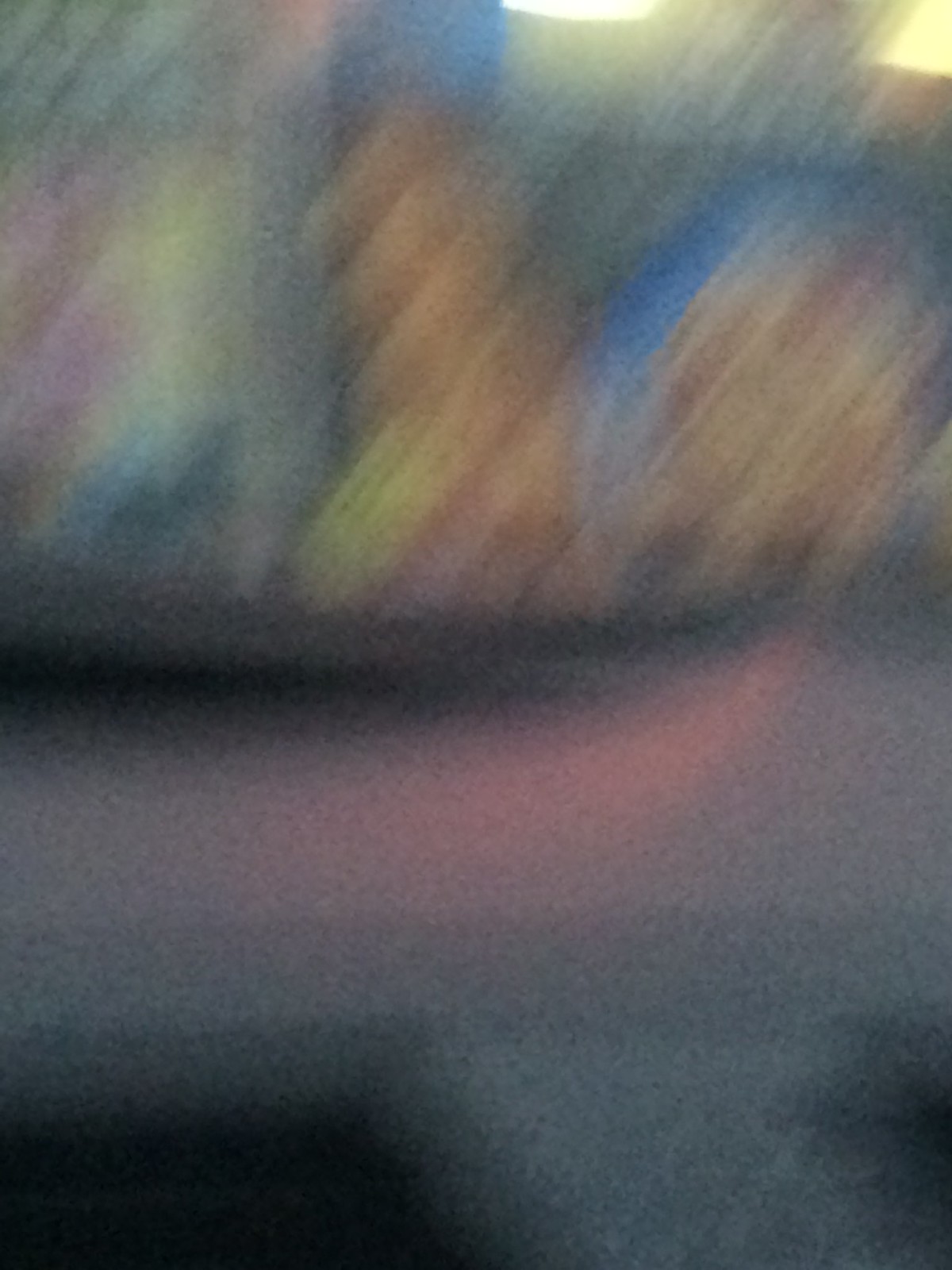A photograph taken through the windshield of a moving vehicle, resulting in a highly blurred image. The lower half of the picture shows a grayish dashboard with a faint pink glow on the right. The bottom left corner is shrouded in darkness. Through the windshield, various indistinct store signs are visible, including an orange-yellow blur in the center, possibly a poster with pink and yellow hues on the left. In the center, there is a hint of blue, while the right side features a mix of blue and orange blurs, further adding to the chaotic colors and shapes indicative of a night-time scene.